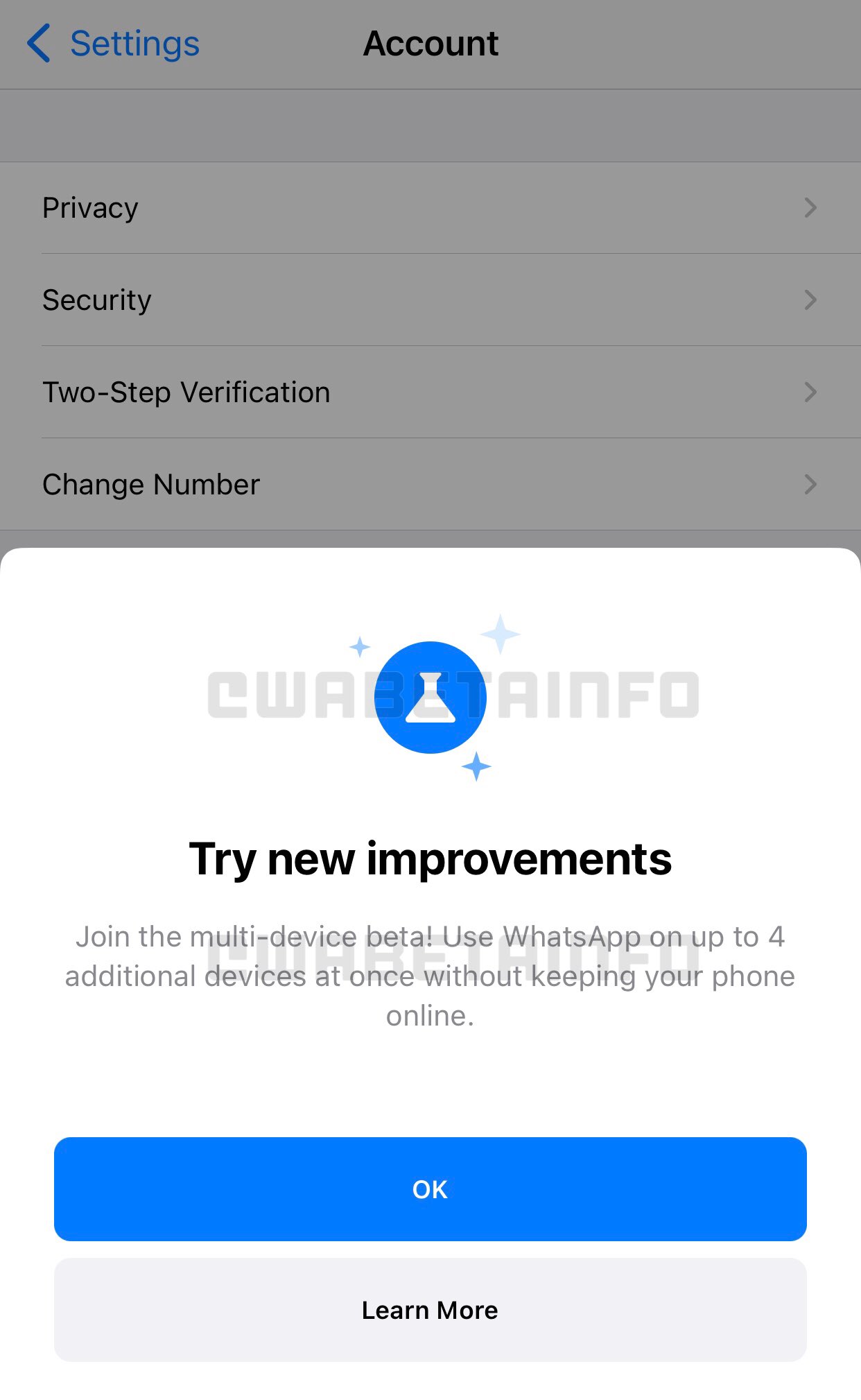The screenshot captures a pop-up message on a mobile device. The pop-up, occupying the lower half of the screen, features a white background with a blue circle containing a white beaker and three blue stars. The top line of the message displays the text "W-A-B-E-T-A-N-F-O" in light gray. The central portion of the message features the prominent, black, centered text "Try New Improvements." Below this, a lighter gray text says, "Join the Multi-Device Beta. Use WhatsApp on up to four additional devices at once without keeping your phone online." At the bottom of the pop-up, there is a blue "OK" button next to a gray "Learn More" button. The background of the screen is grayed out and not interactive, revealing a settings page with multiple options. At the top bar, highlighted in blue, there is a left-facing arrow and the word "Account" in black. Below this, there are menu items including "Privacy," "Security," "Two-Step Verification," and "Change Number," each accompanied by a right-facing arrow, all set against alternating dark and light gray bars.